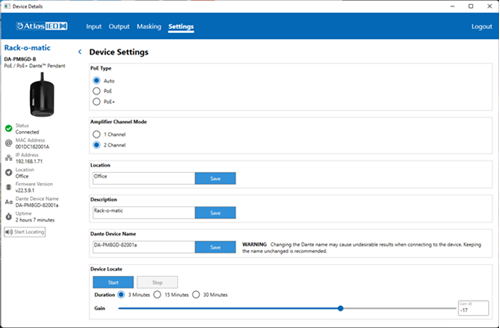The image depicts a user interface of a black device labeled "Rack-O-Matic" in blue text. At the top, a blue bar reads "Atlas and something" (unclear), and the interface features multiple tabs labeled Input, Output, Marking, Making, Unsure, and Settings. Below these tabs, there is an arrow pointing to the left next to the words "Device Settings." 

Several small selectable circles are visible, with the top circle highlighted in blue, indicating it is currently selected. Text associated with these circles is illegible, but one phrase stands out: "one device, two device," with "two device" having a blue circle filled in.

A text box is provided for user input, accompanied by a blue "Save" button. Further down, labeled areas include "Description" or "Descriptives," with another text box for input and an adjacent blue "Save" button. Another section labeled possibly as "Device Name" includes a text box and a "Save" button.

A warning section is noted, though its detailed text is unreadable. Below it, another text line precedes a blue "Save" button, a white "Stop" button, and additional options marked by blue circles and an unidentified slider bar, with text too small to decipher.